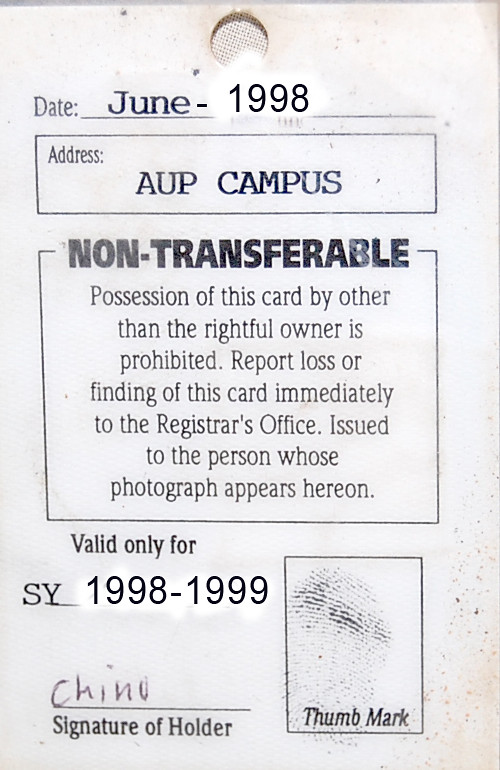This image features an old, somewhat dirty, and stained leaflet issued in June 1998 for AUP campus. At the top is the date, "June 1998," along with a circle punch-out. Below this, the address "AUP campus" is displayed. In the next section, bold black letters declare "non-transferable" and include a notice stating, "Possession of this card by other than the rightful owner is prohibited. Report loss or finding of this card immediately to the registrar's office. Issued to the person whose photograph appears hereon." Further down, it reads, "Valid only for SY 1998-1999," alongside the signature of the holder, "Chino," written in purple ink. Adjacent to the signature is a black-outlined rectangle containing a fingerprint with the label "thumb mark" beneath it.